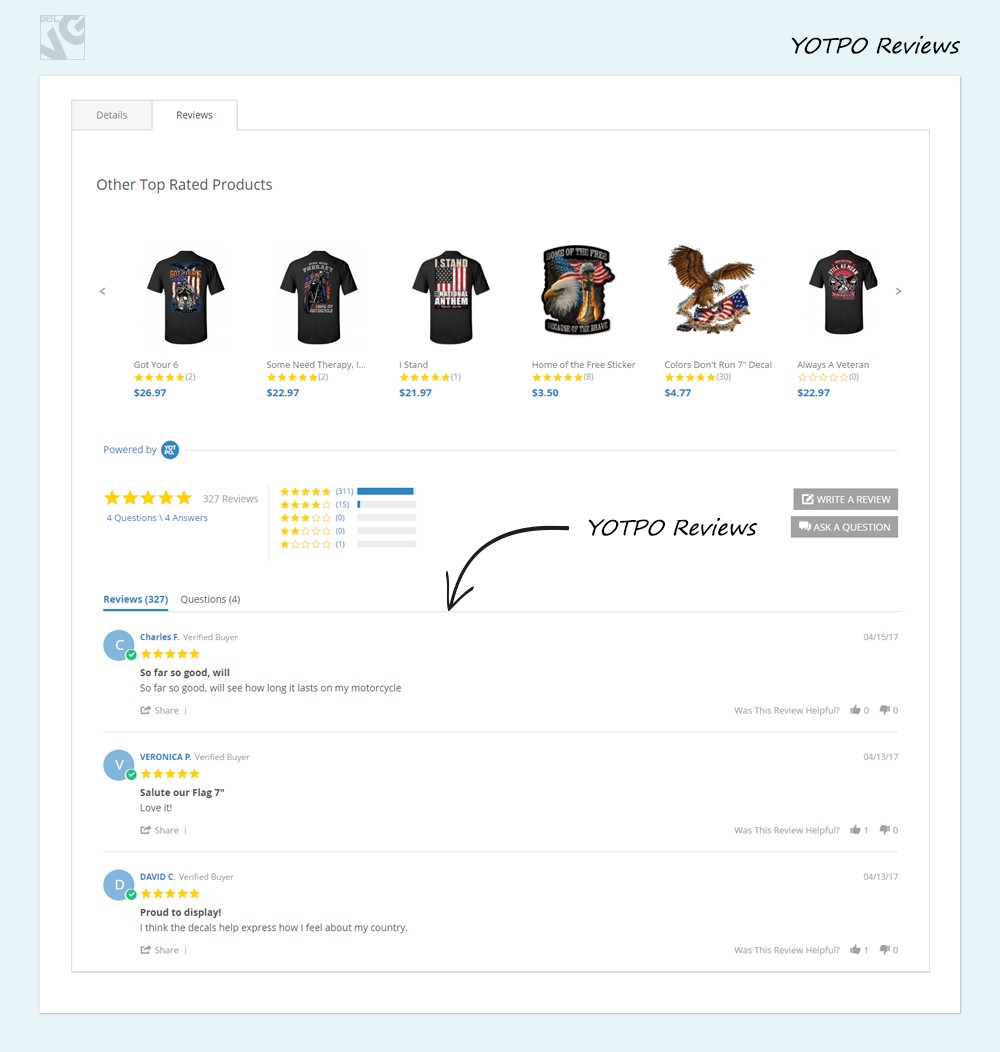This image is from an online shopping website. The outer border of the image is light blue, measuring about half an inch at the top and a quarter-inch on the sides and bottom, while the inner background is white. 

In the top-left corner, there is a small square containing a stylized "V" angled down to the right, followed by a "G" angled similarly, both in black. Next to this square are the black, capitalized letters "YOTPO." To the right of "YOTPO" is the word "Reviews."

Beneath this, there is a thin gray border encasing the entire section. At the top of this border, a gray tab labeled "Details" in black text is displayed, with a white tab to its right that reads "Reviews." Below this header, the section states "Other Top-Rated Products."

The main content area showcases images of three shirts, a sticker, and a decal, followed by another shirt beneath them. Each product image is accompanied by its name, rating (displayed as stars), and the price, which is shown in blue text. Below each price, the text reads "Powered by" followed by a blue circle with the letters "YOT" on top and "PO" underneath.

Further down, there are detailed star ratings, displaying the number of reviews each product has received across five categories: five stars, four stars, three stars, two stars, and one star.

In the center of the image, the text "YOTPO Reviews" is prominently displayed, accompanied by a black arrow pointing left and then downwards. To the right, there are two gray tabs: one labeled "Write a Review" and another labeled "Ask a Question." Below these tabs, the image features three reviews left by customers.